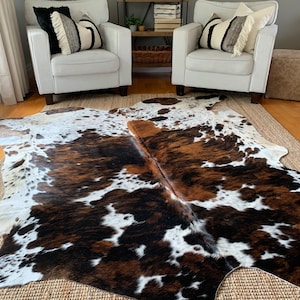The image is set in a cozy living room, showcasing a luxurious, brown wooden floor. Centered on this floor is a distinctive area rug. This base rug is a soft brown hue, providing a warm contrast to the striking, irregularly-shaped animal skin rug draped over it. The animal skin rug, possibly a cowhide, features a captivating mottled pattern of browns, blacks, and whites, with predominantly white sections accented by brown splotches and dark dots along the far edge and left side. Toward the back of the scene, two cream-colored sitting chairs are positioned, each adorned with an array of pillows—three on the left chair and two on the right—all adding layers of comfort and style. A small table or shelf can be seen behind these chairs, holding various items including the base of a lamp, further enriching the cozy and detailed ambiance of the room.